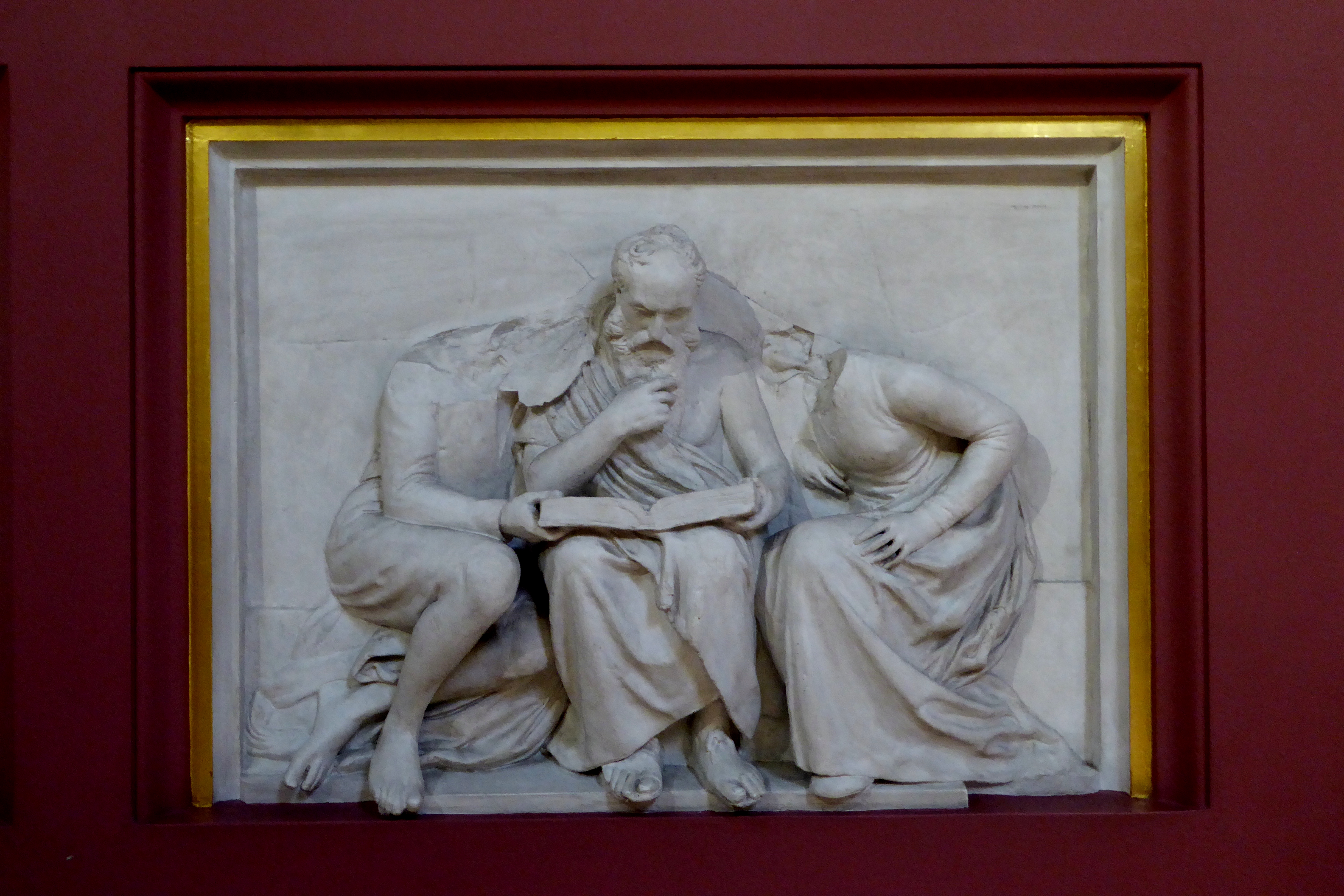The image is a horizontally aligned, rectangular photograph with a maroon-colored background. In the center is a picture frame that blends seamlessly with the background, featuring a maroon wood border and a thin gold interior outline. Within this frame, there is a grayish depiction of a three-dimensional marble statue. This statue portrays a man at the center, who is seated with a thick, open book on his lap, seemingly engrossed in its contents. He wears a toga and sandals, and his right hand thoughtfully strokes his beard. Flanking him are two women dressed in long gowns; their faces are obscured as they lean into the man’s chest and shoulders. The woman on the viewer’s left clutches the book, while the other has her hand resting on her leg, which is crossed. The intricate interplay of their forms makes it appear as though the figures are melded together, emphasizing the sculpture's detailed craftsmanship.